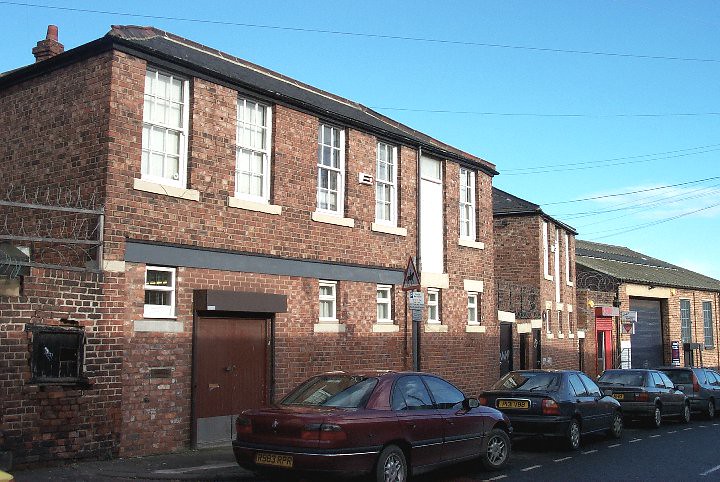This photograph captures a sunny street scene that could be reminiscent of England, depicting a row of brick buildings, mostly two stories high, extending from the left to the right side of the image. The buildings feature white trim and window frames, with smaller windows on the ground floor compared to the larger ones on the upper floor. Some structures have double doors, and the one closest to the foreground has a visible chimney in the upper left corner of the image. The buildings are separated by low brick walls topped with spirals of razor wire, with electrical cables crisscrossing a clear blue sky that boasts sparse, low-lying clouds. In the lower right-hand side of the photograph, a line of four cars is parked along the curb. These cars, all sedans from the 90s or early 2000s, are dark-colored with yellow license plates. The car closest to the foreground is burgundy, followed by a dark green one, then a gray one, and another gray car furthest away. The street appears standard and urban, with the main building featuring a double door and the one furthest back seeming to be an industrial building with a garage opening.